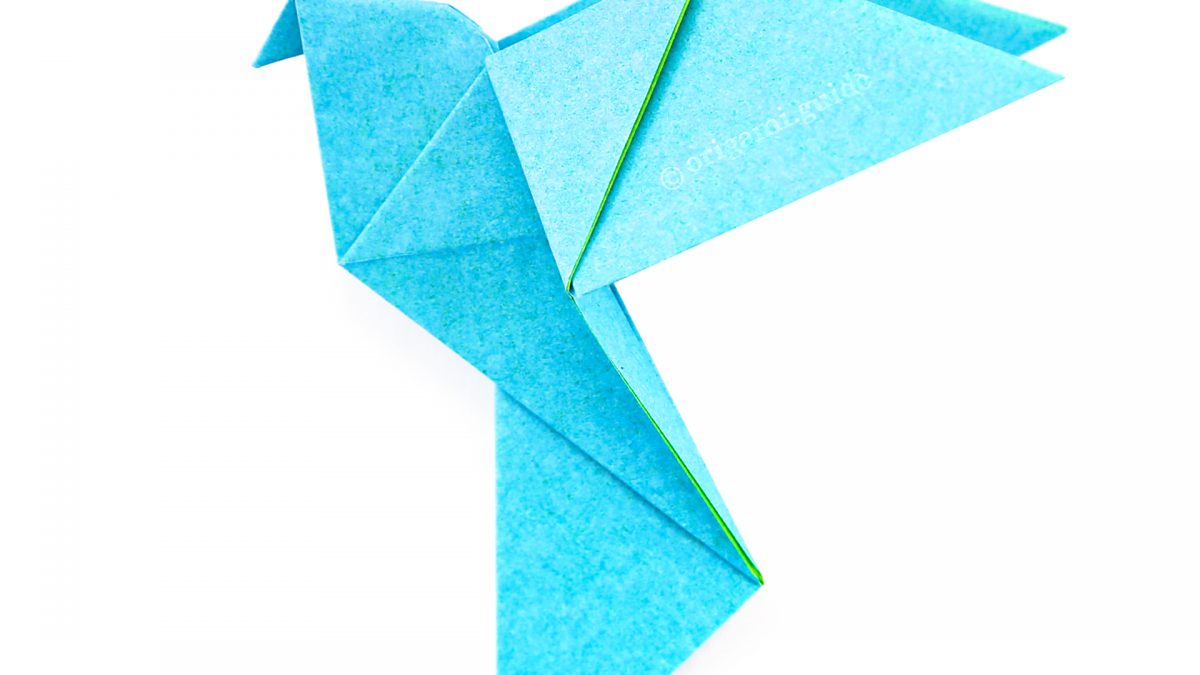The image features a close-up photo of a meticulously folded origami bird made from light aqua blue paper, resembling a dove in flight. The intricate folds and detailed design showcase the artist's skill, though the exact folding pattern remains complex and challenging to discern. The bird sports a beak, body, tail, and two wings, creating a polygonal yet elegant shape. The background is a plain white surface, offering no additional context. Notably, the bird's front wing faintly bears a copyright symbol (©) followed by the text "origami.guide" in lowercase, though this is barely legible. The overall hue of the paper carries a faint resemblance to a light blue jean color, akin to indigo.